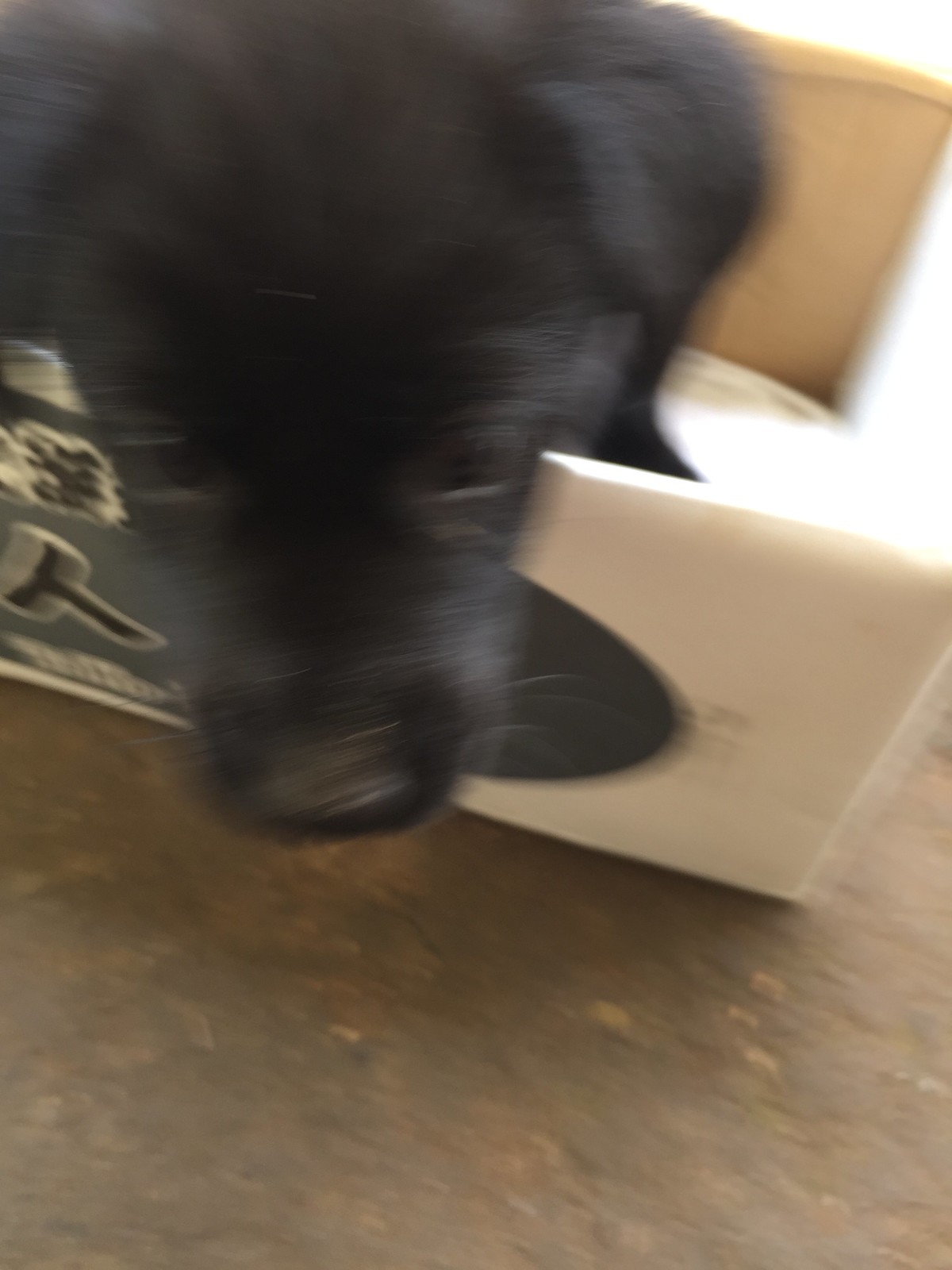The image is a slightly blurry photo of a cute black Labrador puppy appearing to climb out of an off-white box. The dog's entirely black face, including its distinctive whiskers, black ears, and nose, is the central focus of the image. It looks like the puppy is popping out from the top left corner of the box, gazing downward. The box is partially visible and has a potential graphic on the left side and perhaps a Japanese or Chinese character somewhere, alongside a black circle in the middle. The background surface appears to be a solid, brown, rocky or concrete ground, suggesting an outdoor setting. Light enters from the top right, although it does not highlight the puppy significantly. The image cuts off part of the puppy’s head, and it seems there might be a white blanket inside the box, but details remain unclear. Despite the blur, the overall cuteness of the young Labrador shines through.